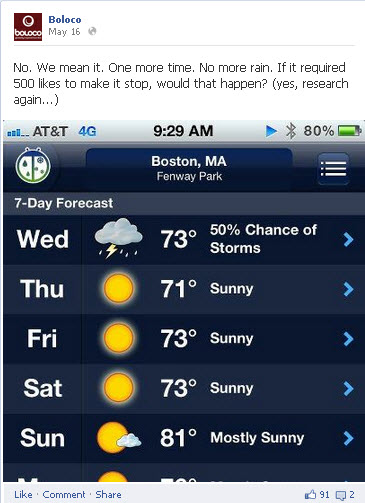**Detailed Caption:**
This screenshot from a public Twitter post by Beloco, dated May 16, features a clean white background typical of the standard Twitter interface. The maroon avatar displays the word "Beloco" in white script. Above the tweet, there is an additional circular icon with a white outline. The text of the tweet reads: "No, we mean it, one more time, no more rain. If it required 500 likes to make it stop, would that happen? (yes, research again)."

Accompanying the tweet is a screenshot of a mobile phone app, indicating it was taken at 9:29 a.m. on an AT&T 4G network with 80% battery remaining. The app shown is a weather forecasting tool, displaying the seven-day weather outlook for Boston, Massachusetts, specifically Fenway Park.

The background of the forecast section is a deep navy blue. It details the weather from Wednesday to Sunday:

- **Wednesday:** Rainy with a 50% chance of storm, high of 73°F.
- **Thursday:** Sunny with a high of 71°F.
- **Friday:** Sunny with a high of 73°F.
- **Saturday:** Sunny with a high of 73°F.
- **Sunday:** Mostly sunny, high of 81°F, depicted with a cloud partially obscuring the sun icon.